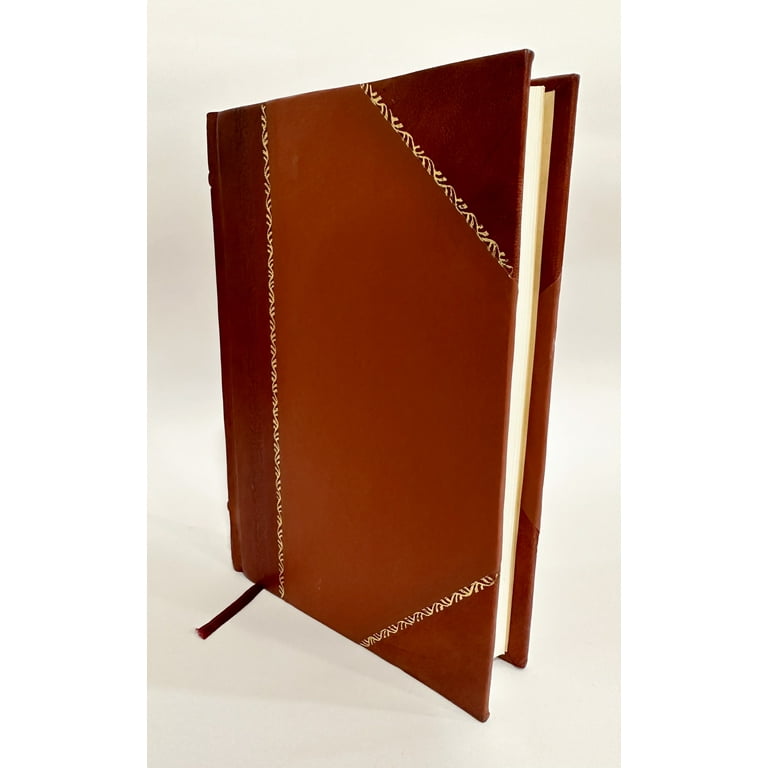This is a close-up photograph of a book standing upright against a white backdrop, creating slight shadows. The book, which appears brand new and not very thick, features a maroon and terracotta red-orange cover with intricate gold embroidery and filigree-style designs. The front cover showcases a central, trapezoid-shaped, light maroon section, bordered by darker maroon sections on the edges and corners. The spine of the book, facing left in the image, is similarly colored but not visible. A dark maroon bookmark ribbon protrudes from the bottom, indicating its function as a page holder. The pages of the book are off-white, contributing to its pristine appearance. The overall design and color scheme suggest it could be an elegant photo album reminiscent of those used in the past.